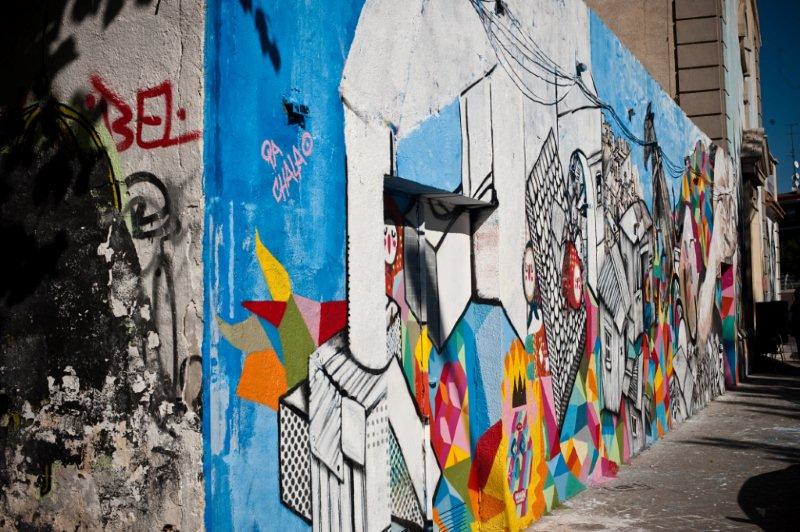The image captures a sunny city street showcasing a vibrant graffiti mural along a large wall. Dominated by geometric and kaleidoscopic patterns in a myriad of bright, vivid colors against a blue background, the artwork displays elements reminiscent of a handmade quilt. The mural includes white and black designs, with some parts bearing distinct signatures, such as a name signed in pink. Toward the far end of the wall, there's a hint of a person holding something near their eyes, although details are obscure due to the distance. Before this, sections of the wall display alternating hues: a segment with "B-E-L" in red on a light gray background, transitioning to "Q-A" followed by "C-H-A-L-A-O" in light pink, and further outlined black and white building imagery. Additionally, the left side of the mural, which appears all-black, could be interpreted as a shadow or darker graffiti. Beyond the main mural, the street continues with a two-story beige building visible down the sidewalk, providing a contrasting backdrop to the intricate and colorful artwork.